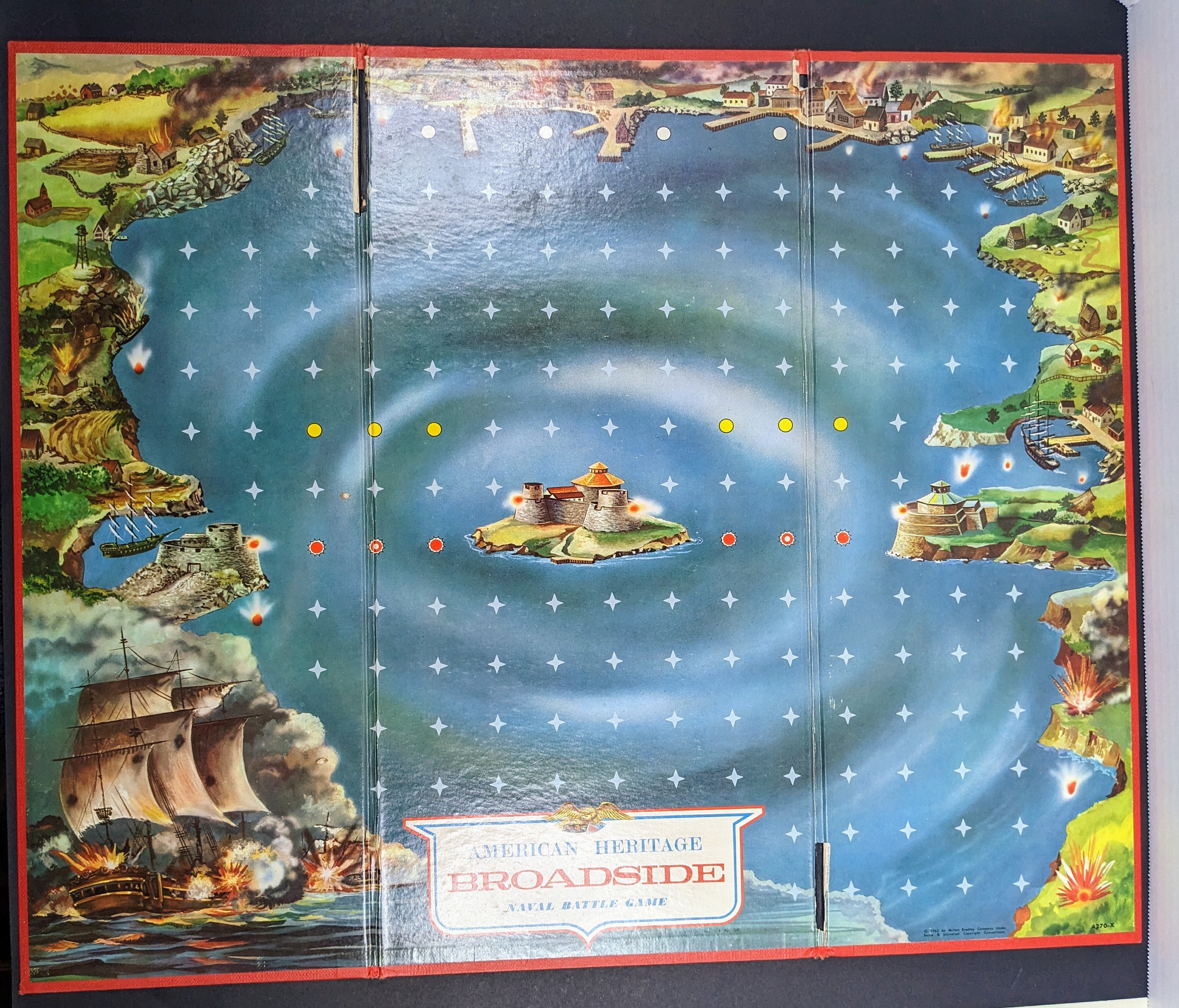The image is a color photograph of the American Heritage Broadside Naval Battle Game package. The package showcases a white-colored logo with an eagle emblem and the game's title written below it. The game board depicted in the image appears to fold up and illustrates a strategic map featuring a large body of water with an island at its center, upon which there is a tower or castle. Surrounding the island are various sections of land forming a sea bay, complete with towns, piers with docked ships, and several noteworthy boats. One prominent boat in the lower left corner seems to be under attack, engulfed in smoke and fireballs. The border of the game package is predominantly red in color, accented with some black portions. The water area on the board is dotted with light blue star shapes, along with yellow and red dots indicating various points of interest or positions where game pieces might be placed.